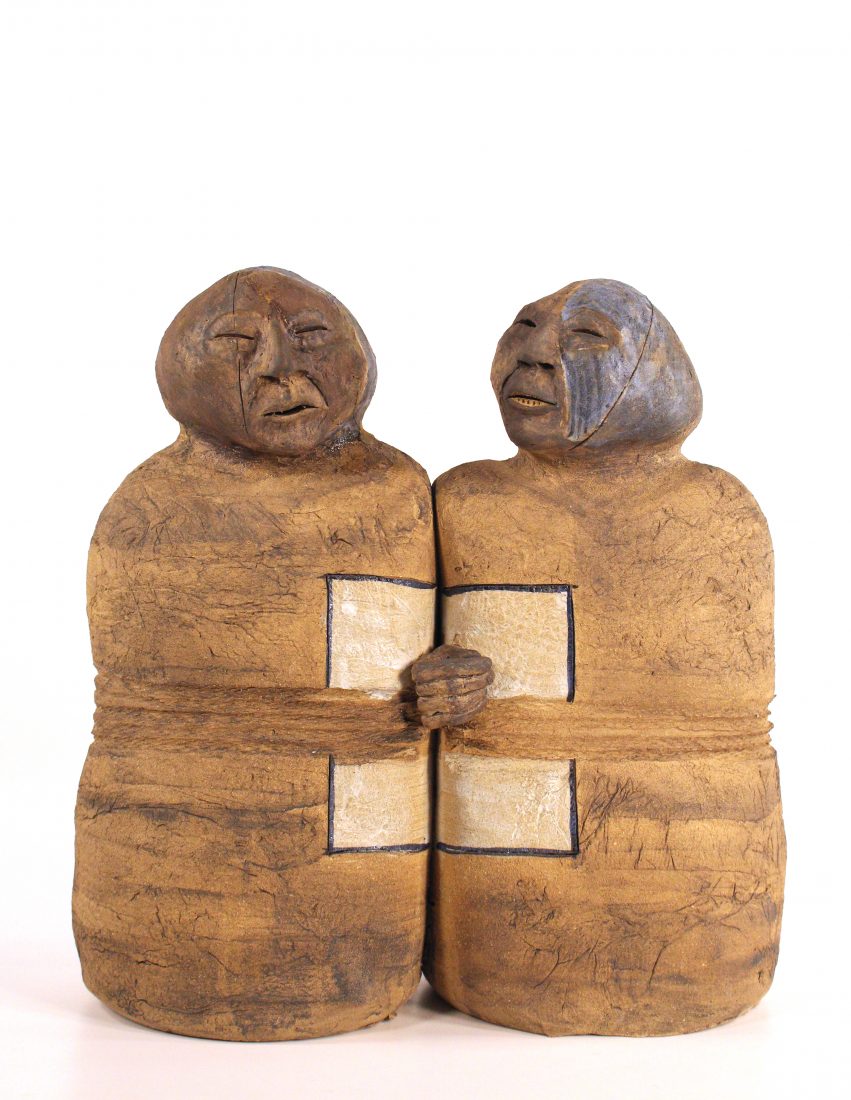The sculpture is an intriguing and rustic abstract piece, appearing to be carved from stone or wood with a beige to dark brown coloration. It features two figures standing side by side, one likely a man and the other a woman, although it's difficult to definitively identify their genders. Each figure has a very primitive appearance with round, rudimentary faces characterized by slit eyes, large noses, and small, slit-like mouths—one figure even appears to be smiling slightly, showing a few teeth.

The bodies of the figures are cylindrical, resembling barrels, with a ridge around the middle. Notably, from their waists, a hand emerges from each figure, and the hands connect in the center, joining the two sculptures together. In the middle of their chests, where their bodies touch, there is a prominent square. This square has a cream-colored interior with a black outline, appearing as though it spans both figures, with one half on each. This detail adds an intriguing focal point to an already captivating piece, making the sculpture both visually and symbolically connected.